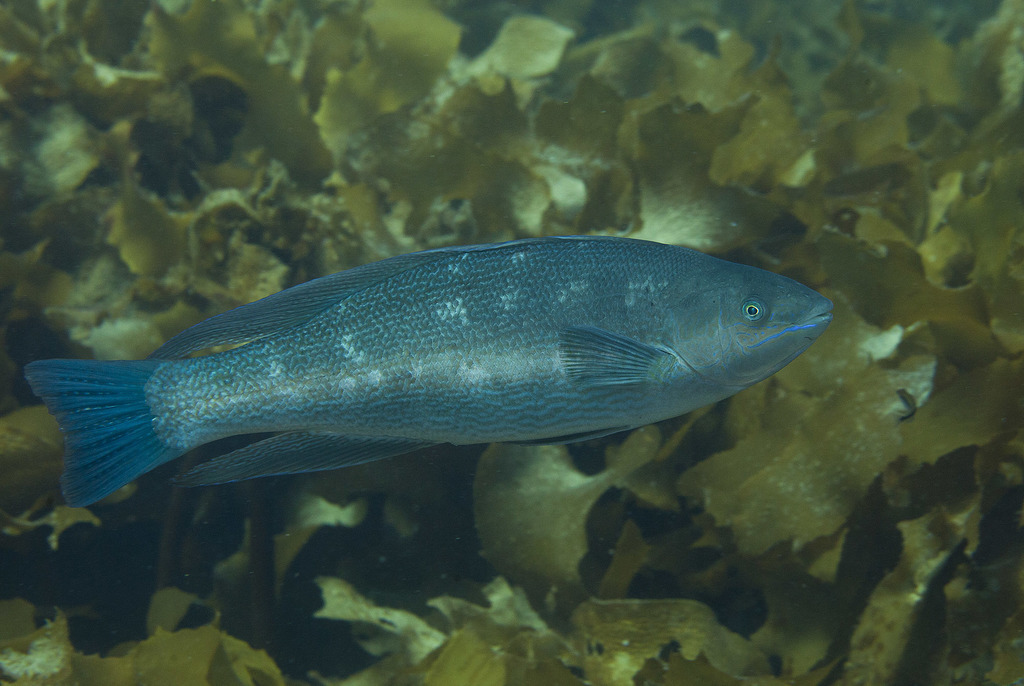A vibrant blue fish with scattered white and lighter blue spots swims gracefully towards the right in the center of an underwater scene. The fish, viewed from the side, has multiple fins: a small one toward the front, one on top of its back, another below, and one at the back. The background is filled with a lush display of greenish-yellow vegetation, possibly underwater leaves or coral, which occupies the entire scene. The vegetation appears denser and darker at the bottom and the top, indicating areas where light penetration is minimal due to the thick plant life. The overall setting suggests a natural aquatic environment, though it’s unclear whether the photograph was taken in the ocean or within an aquarium. The fish's iridescent blue hue stands out beautifully against the vibrant greenery, creating a striking underwater snapshot.